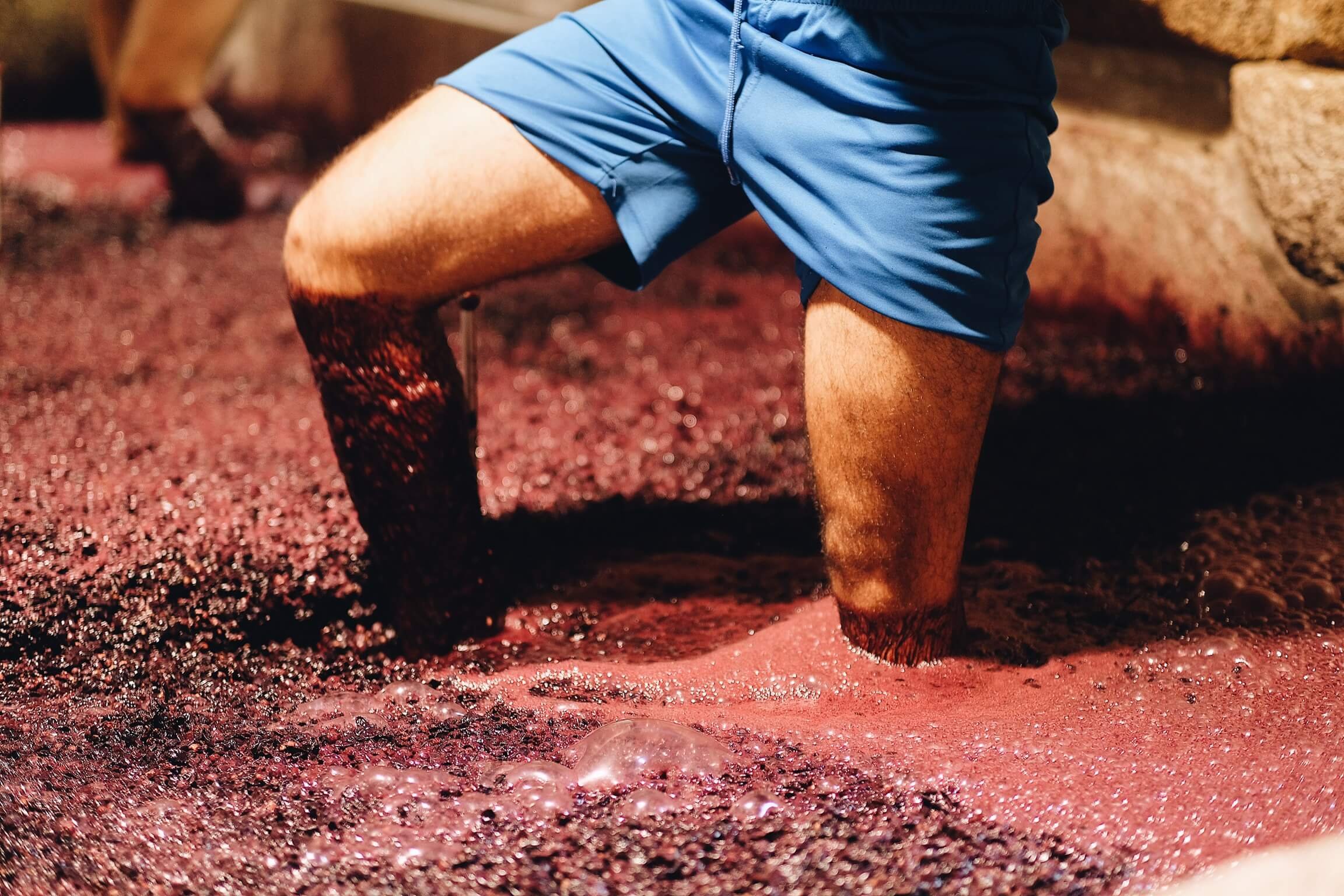This photograph captures the lower half of a man clad in blue shorts, appearing to navigate through a thick, reddish-brown mucky substance that could be mud or clay. His right leg is straight down while his left leg is bent at the knee, seemingly emphasizing his struggle to move. The muck envelops his legs, reaching up to his knees, and appears foamy with some black patches. The backdrop features large light tan rocks, adding a rugged outdoor element to the scene. The image is cropped at the man's waist, focusing solely on his legs and the challenging terrain. No other distinguishing features, such as a date, time, or location, are present in the photo. The colors in the image mainly include shades of blue, flesh tone, tan, black, brown, and various hues of reddish muck.